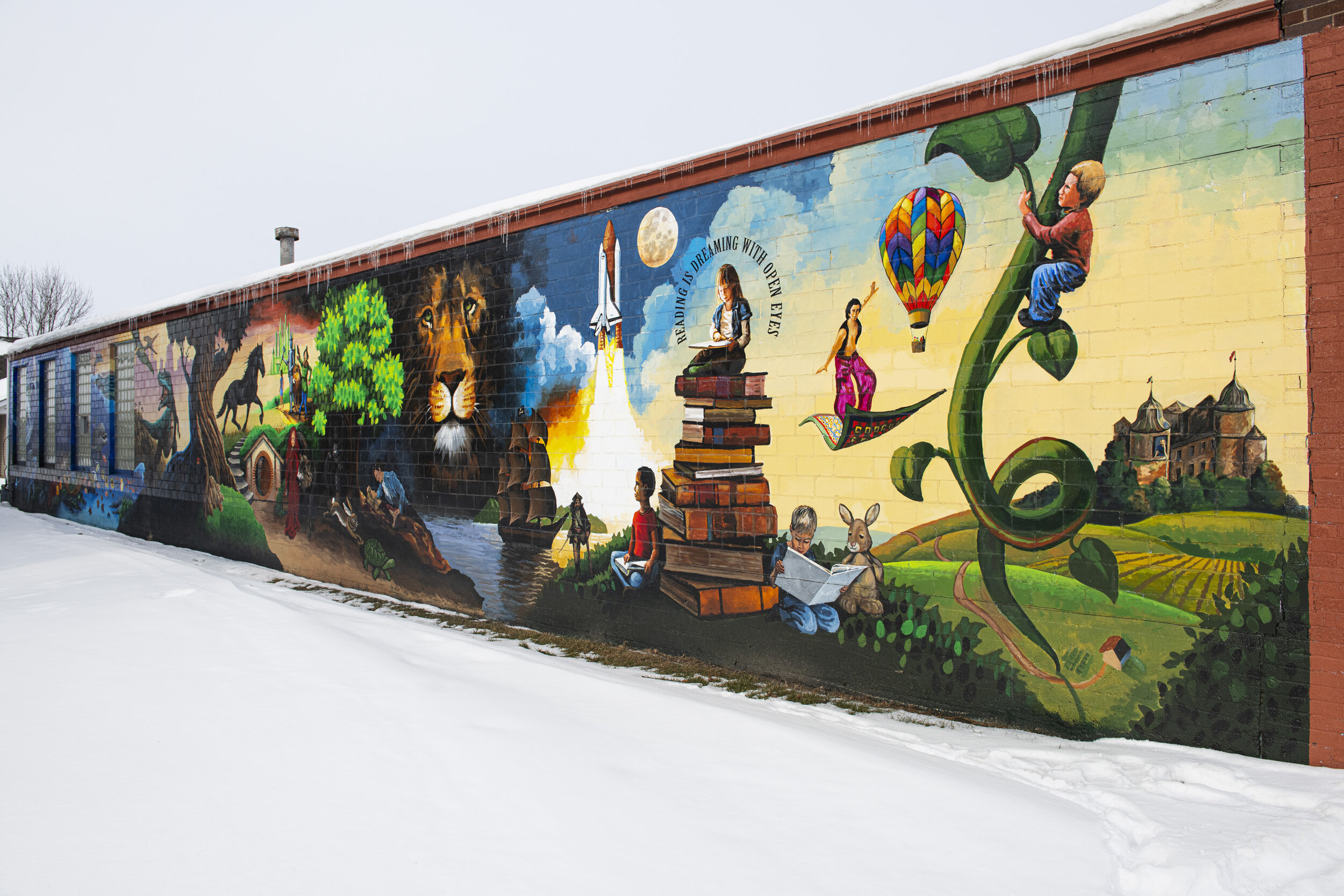This photograph captures a sprawling mural painted on the brick face of a long building, which stretches from the closer right side and tapers off into the distance on the left. It is winter, evidenced by the snow-covered ground, bare tree branches, and icicles hanging from the roof, under a flat gray sky. The mural features a vivid tapestry of various children's tales and significant historical events, covering almost the entire brick surface except for a thin margin that reveals the red brick underneath. 

On the right, Jack from "Jack and the Beanstalk" is seen climbing a giant beanstalk with a castle in the background. Below, Aladdin rides his magic carpet. Moving left, there's a depiction of a hot air balloon and Alice from "Alice in Wonderland" reading a book. Further to the left, there is a young girl sitting atop a stack of books with the text "Reading is Dreaming with Open Eyes" encircling her. Nearby, a rocket ship launches towards the moon. Additional scenes include a lion—possibly from "The Chronicles of Narnia"—a pirate ship sailing, a horse with one hoof raised, galloping past a hobbit-like house set into a hill, and more intricate decorations and windows on the far left. The top and left side of the mural feature various other elements, including water, sails, plants, and a tree, rounded out by a snowy rooftop.